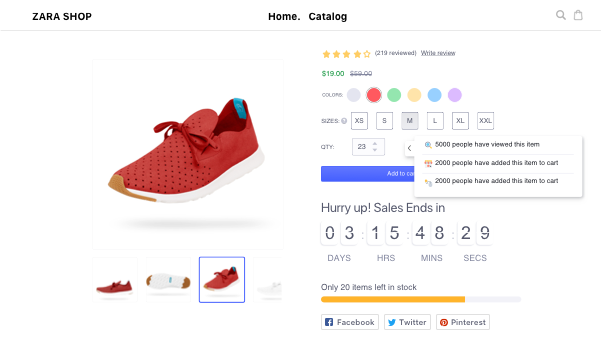The image provides a detailed representation of a retail shopping layout, focusing on a specific product—a shoe. In the top left corner, there is a Zara shop icon. At the center, a handwritten catalog on glass along with a bag is visible, indicating an in-store or online promotion. Featured prominently is a shoe with numerous specific details: it has a brown tip, a white sole, and red shoelaces. The rear of the shoe features a blue lip. The shoe's design includes star patterns—four filled-in stars and one hollow star. 

The product has received 219 reviews, with a highlighted positive review marked in green, mentioning "taller than 19." Various colors are referenced: gray, red, green, yellow, and blue circles, suggesting availability in multiple colorways. 

The coat sizes XS, S, M, L, XL, and XSL are listed, potentially part of the product specifications or related apparel. A stock quantity of 23 is noted. Additional text reveals that 5,000 people have viewed this item, and 2,000 have added it to their cart.

An urgent sales banner in a blue rectangle states, "Hurry up, sales end in 3 days, 15 hours, 40 minutes, 29 seconds," emphasizing time-sensitive availability. There's also a countdown of 29 minutes remaining for another unspecified action.

Social media icons for Facebook, Twitter, and Pinterest are displayed for sharing the product. At the bottom, another red shoe is shown among different varieties, suggesting a broader collection available.